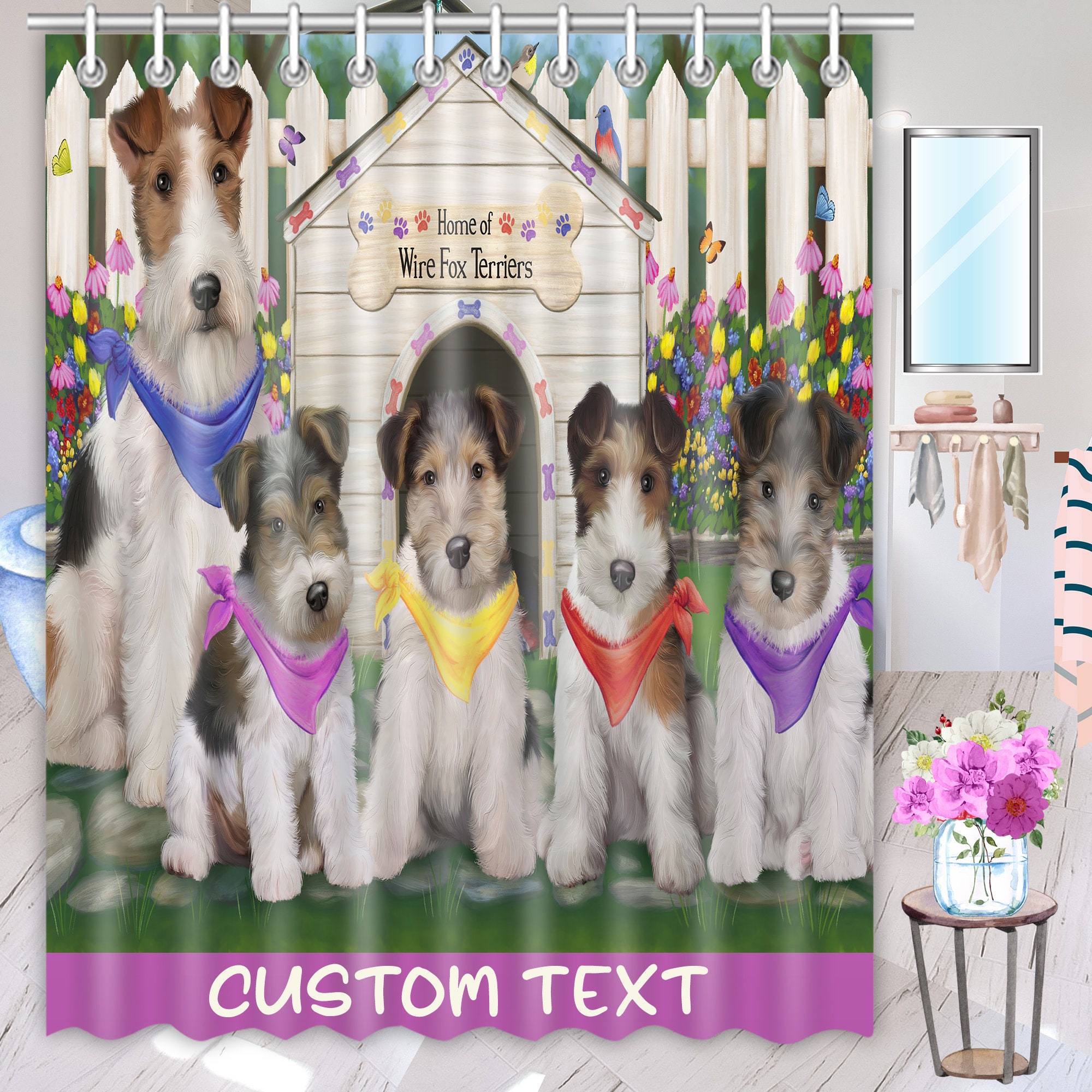The image is a digital illustration designed as an advertisement for a customizable digital greeting card or shower curtain. It depicts five wire fox terriers with white bodies and various face markings, each adorned with a colorful bandana: the largest terrier on the left has a blue bandana, followed by four puppies with bandanas colored purple, yellow, red, and dark blue respectively. They are positioned in front of a white doghouse with a sign shaped like a bone that reads "Home of Wire Fox Terriers." Surrounding the doghouse are multicolored flowers and butterflies, and the entire scene is set against a white picket fence. The backdrop features a bathroom setting with a white wall, a rectangular mirror, a shelf with pegs holding towels, and a small round table with a vase containing purple and white flowers. Below the illustration of the dogs and doghouse, there is a purple band with white text that reads "Custom Text," indicating that the text can be personalized. The image is vibrant and detailed, capturing both the playful essence of the terriers and the cozy, homely environment they inhabit.